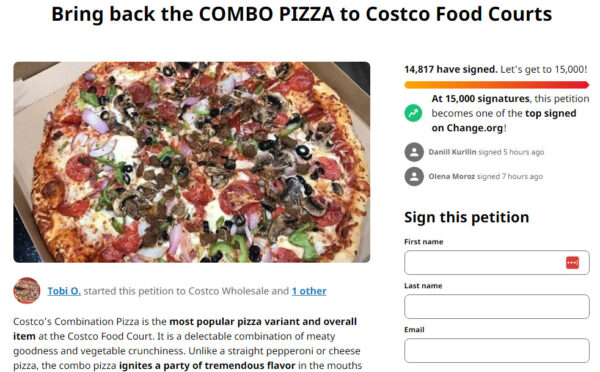A screen capture of a Change.org petition features a clean white background with bold black text at the top stating, "Bring back the combo pizza to Costco food courts." Below the header, there's an image of a savory pizza displaying an assortment of toppings, including sausage, pepperoni, cheese, olives, and green peppers, all nestled in a cardboard pizza box.

To the right of the pizza image, the petition shows progress with a vibrant orange-red bar indicating 14,817 signatures, edging closer to the goal of 15,000. A green circle with a white arrow highlights, "At 15,000 signatures, this petition becomes one of the top signed on Change.org." Nearby, two smaller gray circles notify that Dan Yale Kulgan signed five hours ago and Elena Margoes signed seven hours ago.

Below the progress section, there's a call-to-action in black text: "Sign this petition," accompanied by three blank fill boxes labeled "First name," "Last name," and "Email," with the first box outlined in red.

At the bottom right of the image, a red circle with a pizza icon indicates the petition's creator in blue text, "Toby O started this petition to Costco Wholesale and one other." Following in black text, a brief yet passionate description reads, "Costco's combination pizza is the most popular pizza variant and overall item at the Costco food court. It is a delectable combination of meaty goodness and vegetable crunchiness. Unlike a straight pepperoni or cheese pizza, the combo pizza ignites a party of tremendous flavor in the mouth," with the text cutting off abruptly thereafter.